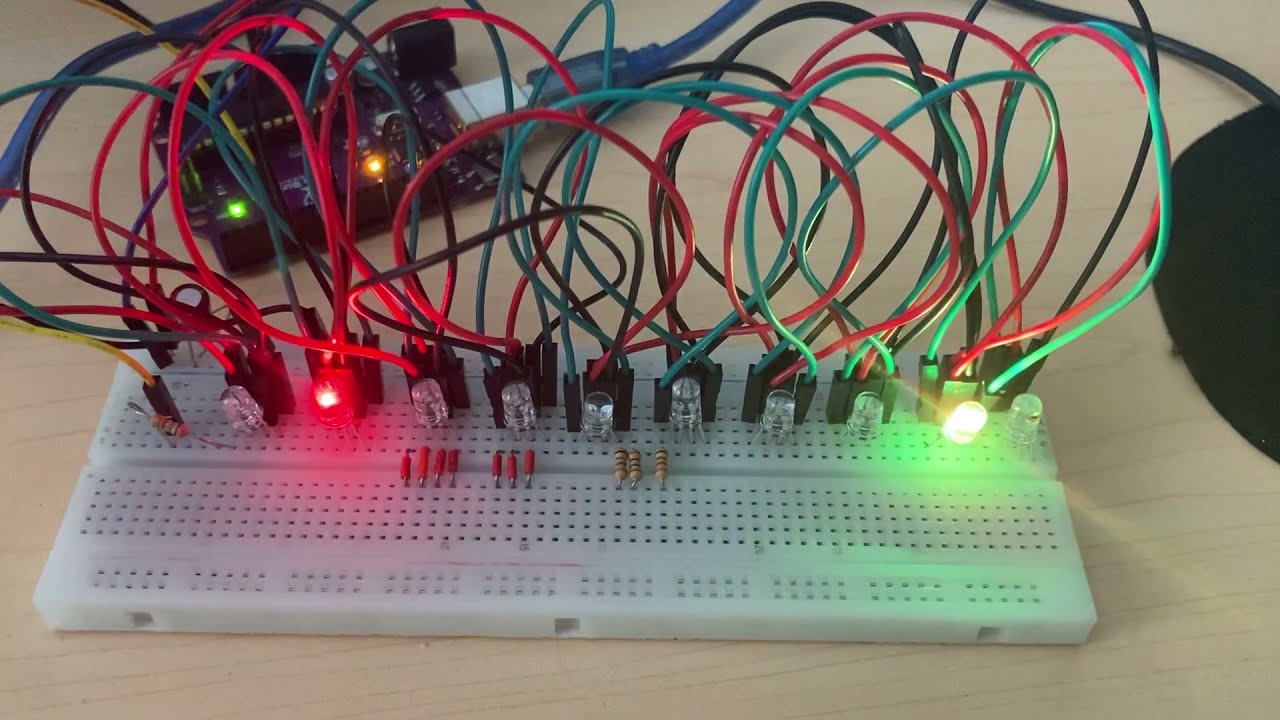The image depicts a plastic white rectangular circuit board with numerous small holes similar to a cribbage board, designed for educational purposes, often found in kits for kids learning about electricity. The board is populated with several black prongs plugged into the holes, each attached to various colored wires—predominantly red, green, yellow, and blue. These wires arc in a slightly disorganized manner across the board, with some connecting to components that seem like resistors or transistors. Notably, there are light bulbs inserted into the black prongs; two of these bulbs are lit, one glowing red and the other white. The circuit board rests on a light tan or beige surface. In the background, there is a black electronic device featuring illuminated green and orange lights, with a blue cord connecting it to the circuit board setup.